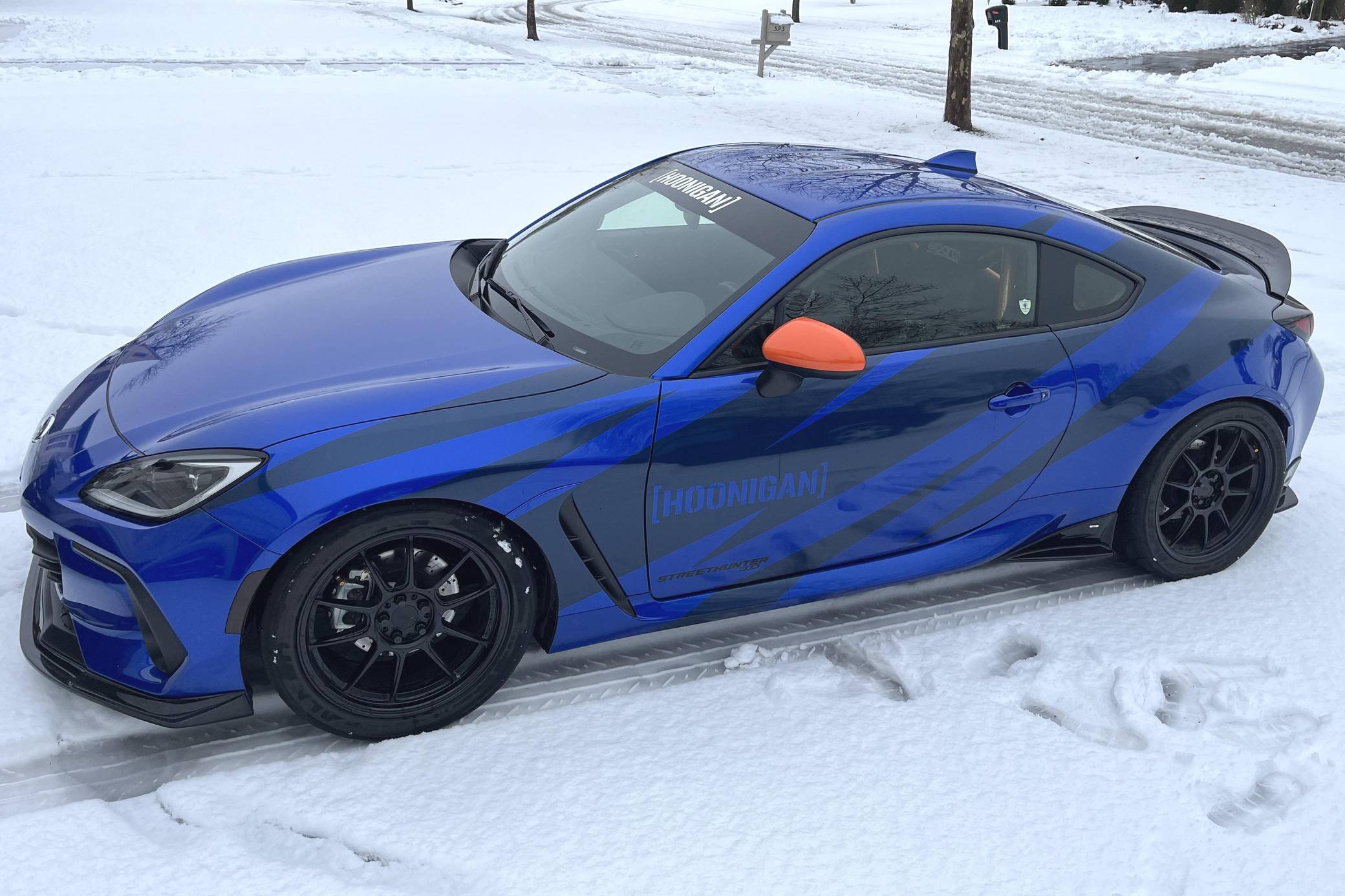This photograph features a striking, gleaming blue sports car parked in a snowy driveway within a residential area. The vehicle, characterized by a neon blue hue with dark, irregular diagonal stripes accented with lightning bolt designs, proudly displays the word "Hoonigan" in blue font across one of the dark stripes on the driver's side door. The car has sleek black tires with black spokes and an eye-catching orange side mirror. A black spoiler is fitted on the rear of the car. The pristine snow surrounding the car is churned up by tire tracks, indicating the car may have been recently parked. Footprints are visible around the vehicle, most likely from someone exiting the car. In the distance, you can see a street lined with mailboxes and a tree or utility pole, with the snow on the street showing signs of vehicle pass-through.